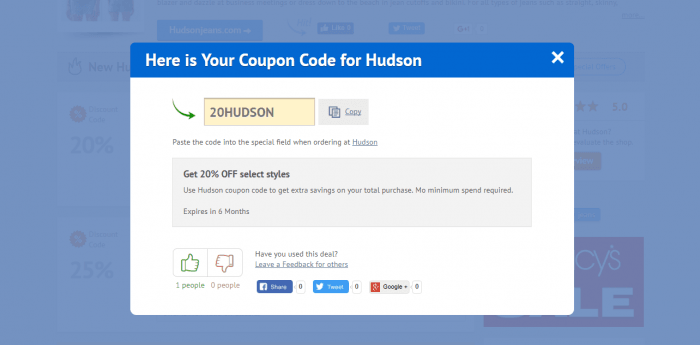The screenshot captures a webpage featuring an active pop-up menu overlay. The background of the website is obscured by a semi-transparent light purple filter, making it difficult to discern details. The focal point of the image is the pop-up menu, designed to provide a promotional coupon code for Hudson.

At the top of the pop-up, there is a dark purple bar with a white font that reads "Here is your coupon code for Hudson." In the upper right corner of this bar is a small white "X" button for closing the pop-up. 

Below the header, the main body of the pop-up is contained within a white rectangle. Positioned at the top of this section is a yellow-highlighted field with a red arrow pointing towards it. Inside the field, in gray font, is the coupon code "20HUDSON." Adjacent to the coupon code is a gray button labeled "Copy."

Underneath the field, instructions in black text encourage users to "Paste the code into the special field when ordering at Hudson."

Further down, there is a gray rectangle with a promotional message in black text explaining the coupon's details: "Get 20% off select styles. Use Hudson coupon code to get extra savings on your total purchase. No minimum spend required, expires in six months."

At the very bottom of the pop-up, there are interactive icons for feedback, including a thumbs-up and a thumbs-down. One user has given the pop-up a thumbs-up.